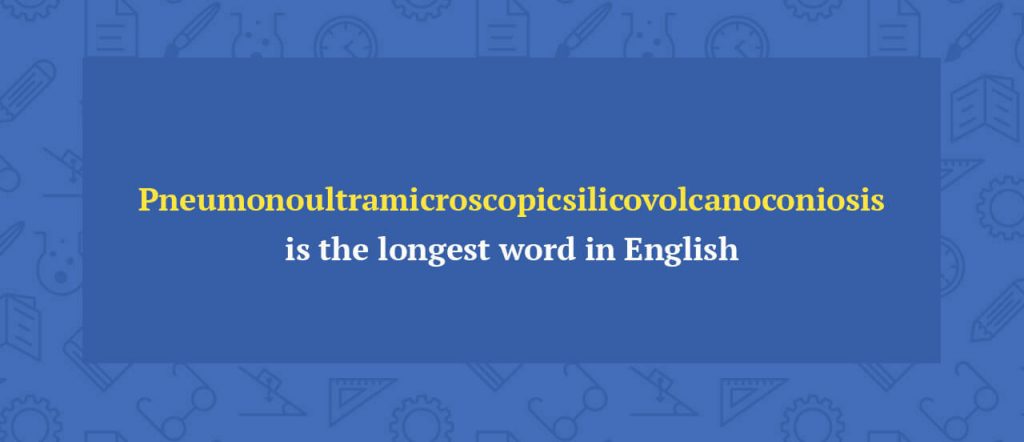A Canva-designed Instagram graphic features a visually appealing dark blue background adorned with scientific elements such as gear pieces, rulers, glasses, clocks, flasks, and books, evoking a scholarly atmosphere. Centered prominently is a darker blue rectangle with yellow text that reads: "Pneumonoultramicroscopicsilicovolcanoconiosis is the longest word in English."